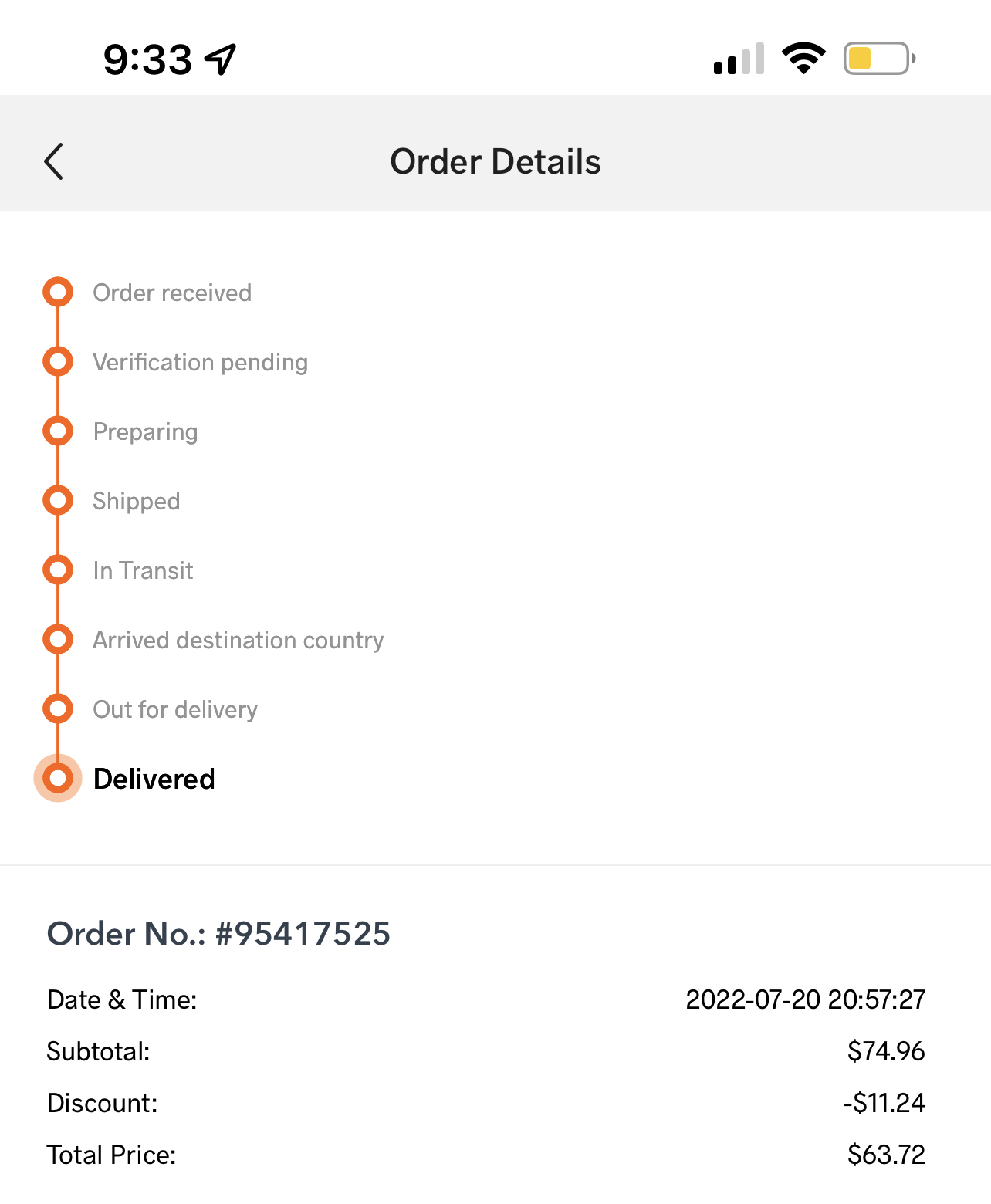This detailed screenshot displays an order confirmation on a smartphone. The top section of the screenshot shows the current time as 9:33, with an arrow pointing upward towards the right. On the right side, the user's phone status is visible, indicating a cellular signal strength of two out of four bars, Wi-Fi signal, and the battery level.

Directly below this status bar is a gray bar labeled "Order Details." Beneath this bar are several red circles connected by lines running down the left side of the screen, each representing a stage of the order process. To the right of these circles, in black lettering, the stages are listed sequentially as: "Order Received," "Verification Pending," "Preparing," "Shipped," "In Transit," "Arrived at Destination Country," "Out for Delivery," and finally, "Delivered," which is highlighted to show completion.

Below this tracking chart, a gray line separates it from additional details. The order number is noted as 954-17525, with the date and time of the order listed as July 20, 2022, at 20:57:27. The subtotal of the order is $74.96, with a discount of $11.24 applied, resulting in a total price of $63.72. Additionally, there is a back arrow on the left side of the "Order Details" bar to navigate back into the app.